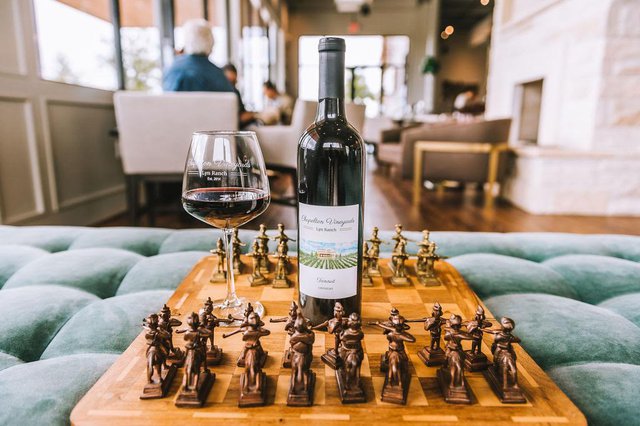The image showcases a horizontally aligned rectangular picture centered on a detailed wooden chessboard positioned atop a green, tufted cushion that resembles sections of a couch or bench. The chessboard is intricately designed with alternating light and dark wood squares. On the closer side, dark brown wooden chess pieces, each with rectangular bases and carvings resembling people, are arranged, while the opposite side features green pieces. A wine bottle with an indistinct white label stands in the middle of the chessboard, accompanied by a partially filled wine glass with some white print, possibly reading "something ranch," located to the left of the bottle. The setting appears to be a cozy, possibly cafe-like environment, with soft cushioned seating and a mix of white and brown chairs. Several people are seated in the slightly out-of-focus background, engaged in quiet conversations. To the upper right, a white stone fireplace with a raised hearth adds to the ambiance, while large glass windows are partially visible in the background, allowing natural light to enhance the scene.